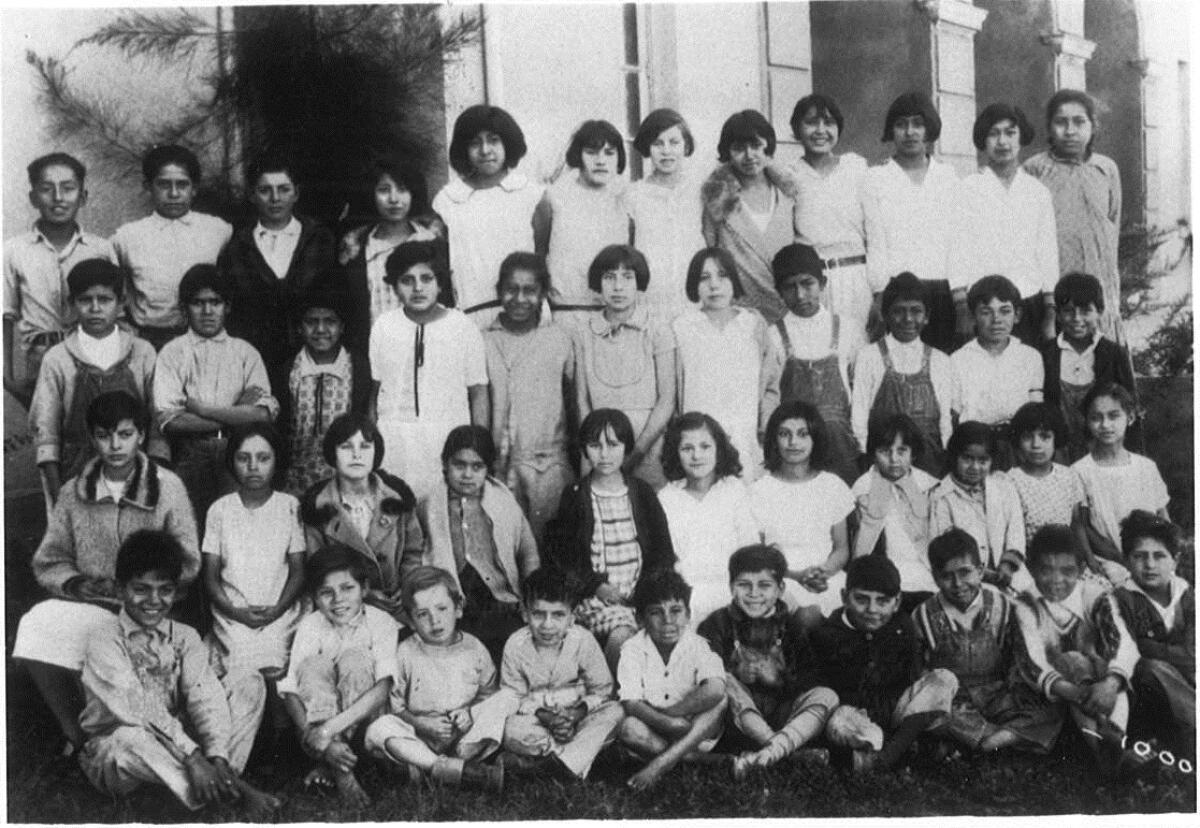The image is a horizontal, rectangular, black-and-white photograph capturing a class portrait of school-aged children. The group is organized into four rows, with the younger children sitting in front and the older children standing in the back. The children, both boys and girls, represent various ages and seem to belong to different nationalities and ethnic groups, including white and possibly Native American. They all have dark hair, and about half of them are smiling. The attire is diverse, with boys wearing short pants, jackets, and overalls, and girls in dresses. No one is wearing hats. 

In the background, there is a white building with no visible signage, accompanied by a wispy tree. At the far end of the photo, it appears there may be a teacher. The photograph has an old-fashioned feel, emphasizing its historical context.